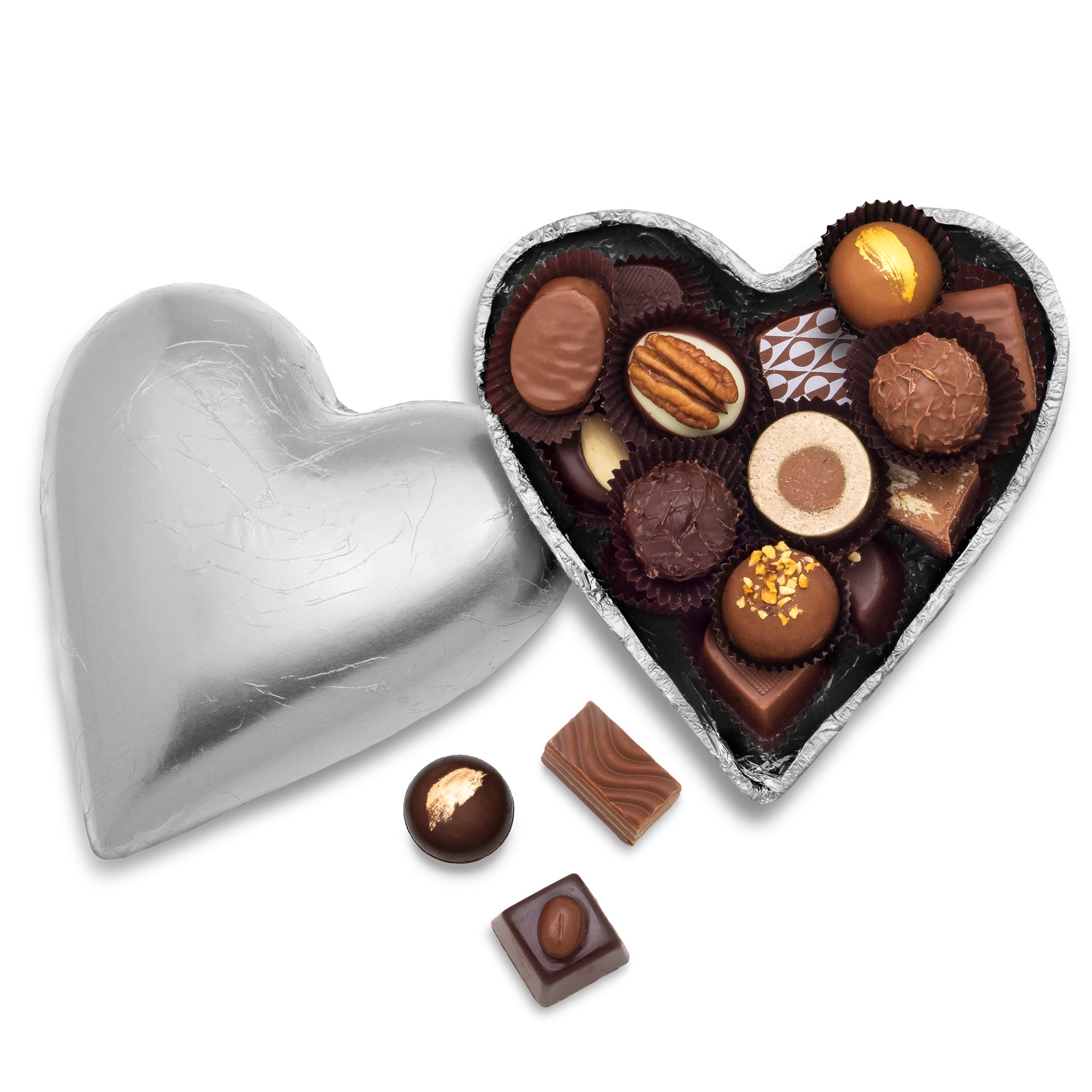This image features a heart-shaped silver box, open to reveal an assortment of brown chocolates in varying shades from light to dark. Inside the box, chocolates are arranged neatly, some wrapped in brown cupcake liner-like paper and others decorated with toppings, such as a pecan. The chocolates come in different shapes; some are round, one is almost nut-shaped, and all showcase intricate designs. The box’s lid lies to the left of the open base, and between them, resting on the white background, are three additional chocolates. These external chocolates include a dark brown circle, a rectangular piece with a swirl design, and a square with a rounded nut decoration on top.